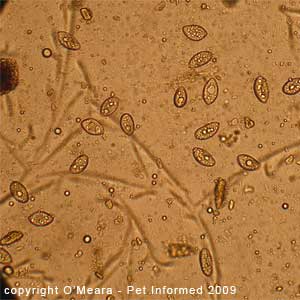This is a small, square image with a tan to medium brown background, resembling a view under a microscope. The image features numerous ellipsoid or seed-shaped structures distributed throughout the frame, about 20 in total. These structures have a dark, well-defined outline and contain lighter, nearly white circular areas inside, along with smaller dots scattered across the background. Additionally, darker brown lines reminiscent of tree branches traverse the image, with some of the ellipsoid shapes aligning with these lines. There is no border around the photograph, and in the lower left corner, it reads in white text, "Copyright O'Meara - Pet Informed 2009".